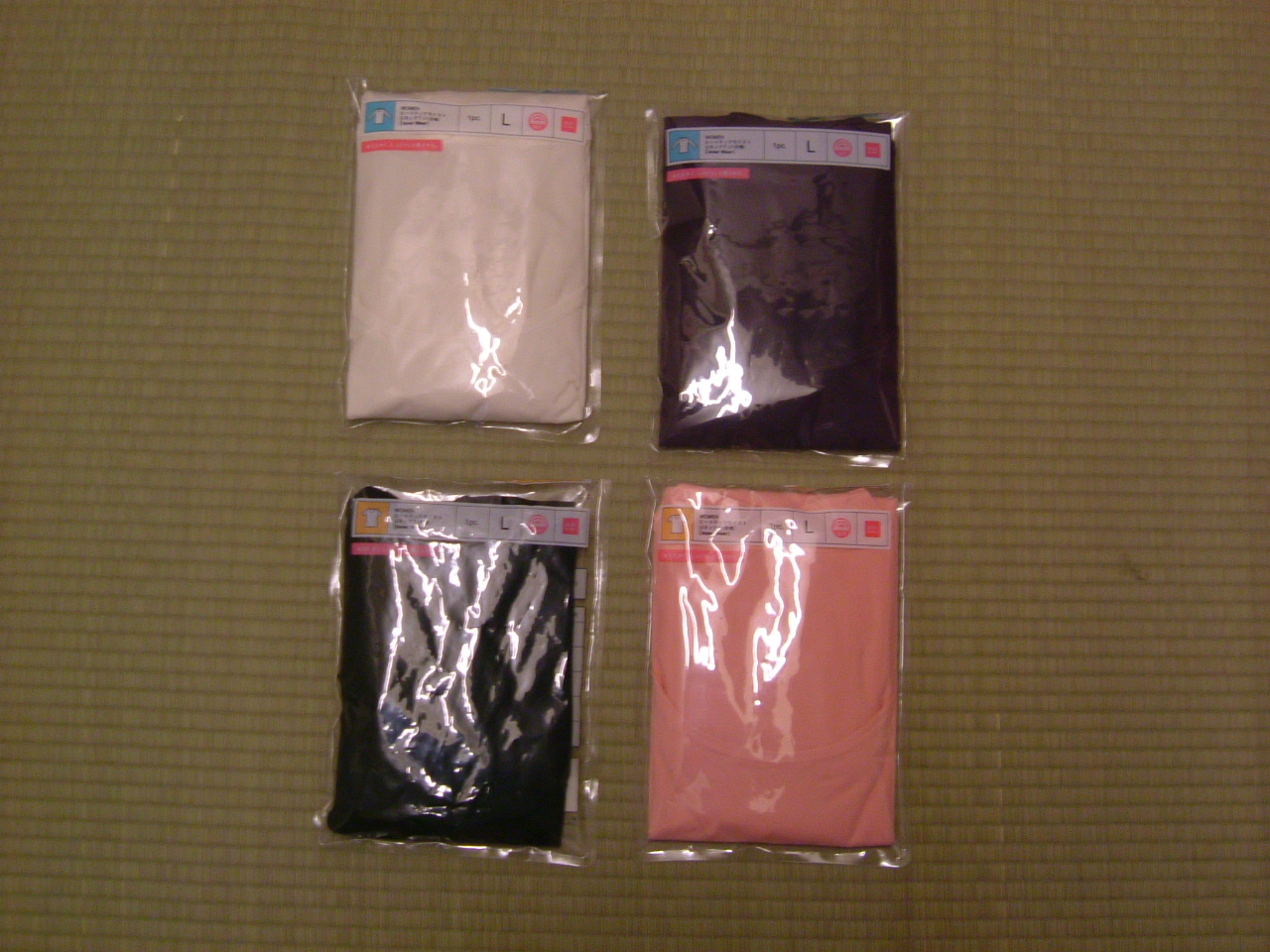This photograph captures four folded t-shirts inside their original shiny plastic packaging, neatly arranged in a 2x2 grid on a tan-colored woven tatami mat. The top left package contains a white long-sleeved t-shirt, while the top right holds a dark brown (possibly black) long-sleeved t-shirt. The bottom left package also has a black short-sleeved t-shirt, and the bottom right features a pink short-sleeved t-shirt with the collar slightly visible. Each package has a size 'L' label at the top, accompanied by a square symbol indicating either long sleeves (blue square) or short sleeves (orange square). The plastic bags reflect light, creating noticeable lines and squiggles on their surfaces. Japanese text, which is unreadable, is also present on the packaging.